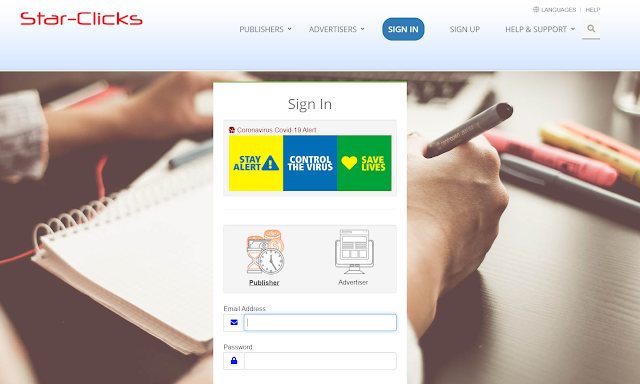The image showcases a website interface with a distinct red header displaying the text "StarClicks" in bold capitals and hyphenated. Positioned in the upper right corner of the page are the words "Languages" and "Help."

Below this, a lighter blue background frames the main navigation menu, which includes categories such as "Publishers" and "Advertisers," a blue tab labeled "Sign In" in white font, and options for "Sign Up," "Help and Support," alongside a magnifying glass icon for search functionality. Apart from "Sign In" and "Sign Up," all menu items feature drop-down options.

The central section of the page is adorned with a graphic illustration. It depicts a workspace setup with a table or desk. A person's forearms and hands are visible, engaged in writing in a notebook with their right hand, accompanied by several pens and colored pens scattered on the table. Adjacent to this scene, a prominent banner text reads "Sign Up," followed by a "Coronavirus COVID-19 Alert" in striking red letters.

Beneath the banner are three vividly colored squares. The first square is bright yellow with blue text that reads "Stay Alert." The second square is blue with white text stating "Control the Virus." The third square is green with yellow text that says "Save Lives" and presents a yellow heart icon.

Further down the page, a rectangular section contains icons symbolizing various time measurements like an hourglass and a clock, labeled "Publisher." A computer graphic with a newspaper emerging from it is labeled "Advertiser." Towards the bottom, fields are provided for entering an email address and a password.